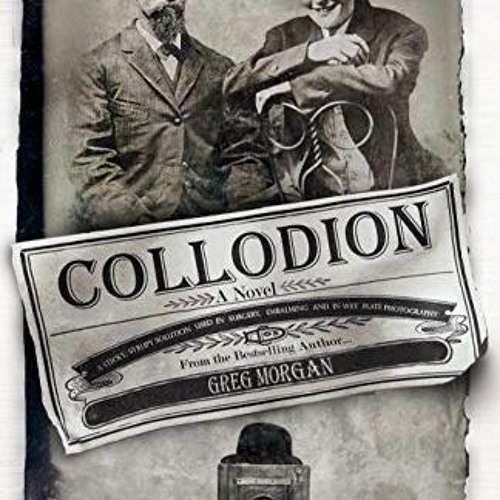The image appears to be a black-and-white photograph with a vintage aesthetic, reminiscent of an old-timey advertisement or a book cover. Dominating the picture are two well-dressed men from the 1800s, their heads partially cropped out of the frame. The man on the left sports a short beard and wears a jacket and tie, while the man on the right sits on a parlor chair turned backwards, facing outwards with a broad smile. The composition suggests a formal yet relaxed setting. Across the center of the image is a banner reading "Collodion, a novel from the bestselling author Greg Morgan," styled like an antique medicine label. Below this, at the bottom of the image, an object that might be a bottle or a table with a hat can be partially seen. The overall effect is one of nostalgic charm, blending elements of historical depiction with literary promotion.